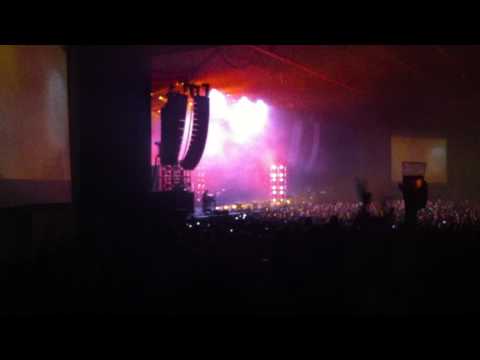The photograph captures a vibrant concert taking place in an indoor venue. The distant stage is illuminated with a blend of magenta, white, and yellow lights, creating a colorful atmosphere. A hazy, smoky effect adds to the dramatic lighting on stage. Amongst the lighting setup, there's a red powder effect being ejected from the top, enhancing the visual spectacle. Prominent features on stage include a stack of speakers and two large screens displaying yellow images, positioned on either side for the audience's convenience. The crowd, densely packed, extends far into the distance, with many attendees holding up phones to capture the moment. Although the image is somewhat blurry, it highlights the magnitude of the event with possibly up to a thousand fans in attendance. Intrusive elements such as a black pillar on the left and the dark area at the bottom of the photograph suggest that the shot was taken from a less optimal vantage point, possibly from the far back right side of the venue. The overall ambiance of the scene is electrifying, albeit difficult to discern individual details due to the combination of lighting effects and distance.